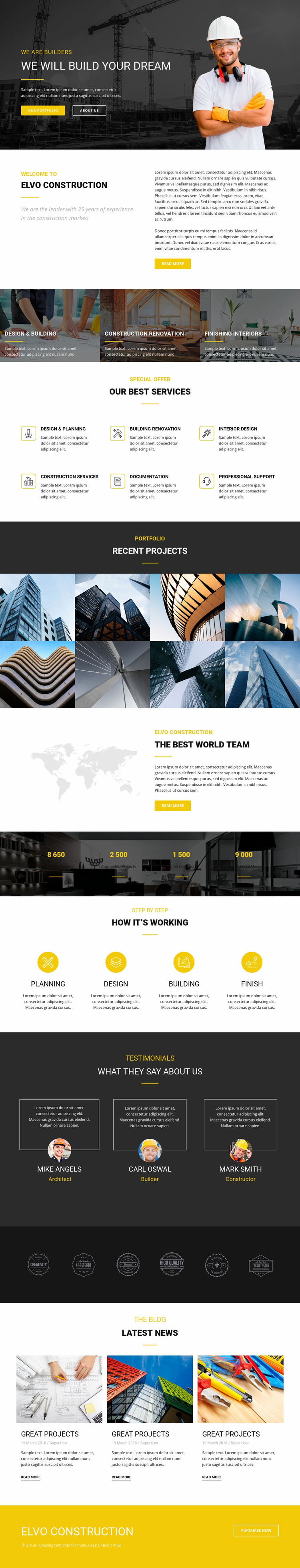Vertical rectangular image illustrating a construction company's website. The elongated layout makes much of the text illegible, but clearly visible at the top in bold, white capital letters are the words: "WE WILL BUILD YOUR DREAM." To the right, an image features a construction worker seen from the waist up. The worker is wearing a white hard hat, a white t-shirt, and yellow gloves, with arms crossed confidently. They also appear to be wearing noise-canceling headphones.

Below this section, various website categories are partially discernible. The first section titled "Our Best Services" lists six distinct services, although the specifics are unreadable. The next notable section, "Recent Projects," showcases a series of project images arranged side by side, followed by "The Best World Team" and "How It's Working." Toward the bottom of the image, the "Latest News" section displays three news stories arranged side by side. Overall, the image captures a visually appealing, comprehensive layout designed to market the construction company's services, recent work, team, and industry news.